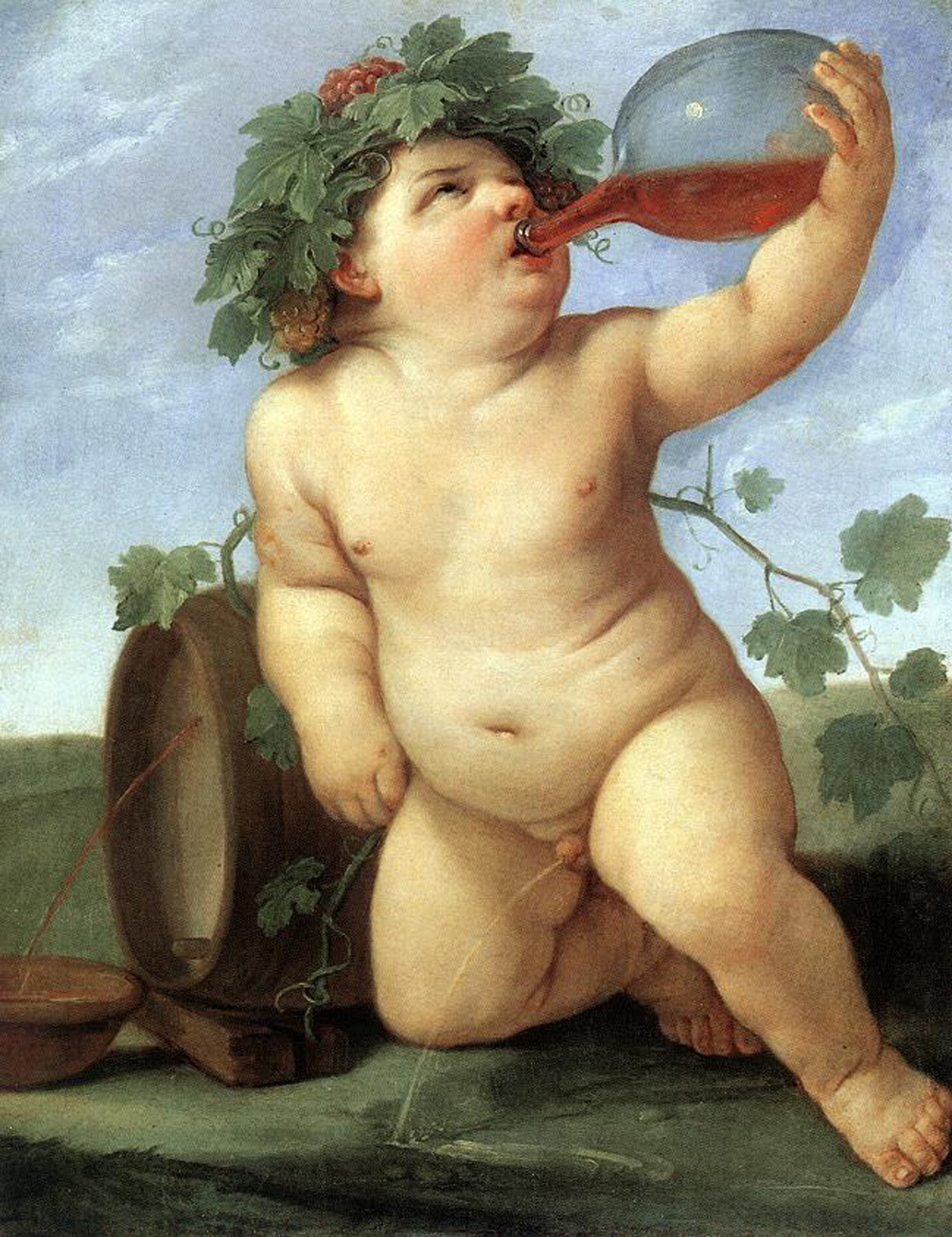This vertical rectangular painting features a chubby, naked baby boy positioned centrally and prominently within the artwork. The child, who has plump arms, legs, and a rounded stomach, is portrayed drinking a red or brown liquid from a wide-based jug or glass flask with his left hand raised above him. The baby gazes upward towards the upper right, wearing an ornamental wreath of green leaves and grapes or berries on his head. With his right arm, he leans against a brown barrel, which has a hole leaking liquid into a brown bowl below. Notably, the baby is urinating, and the stream hits the ground. Surrounding the child, the ground is depicted in shades of grayish-green, and a green vine is visible behind him. The background blends into a sky filled with blue and white hues, featuring clouds, creating a serene atmosphere. The painting appears richly detailed and is composed with numerous vivid colors, including gray, white, green, red, orange, tan, and brown.